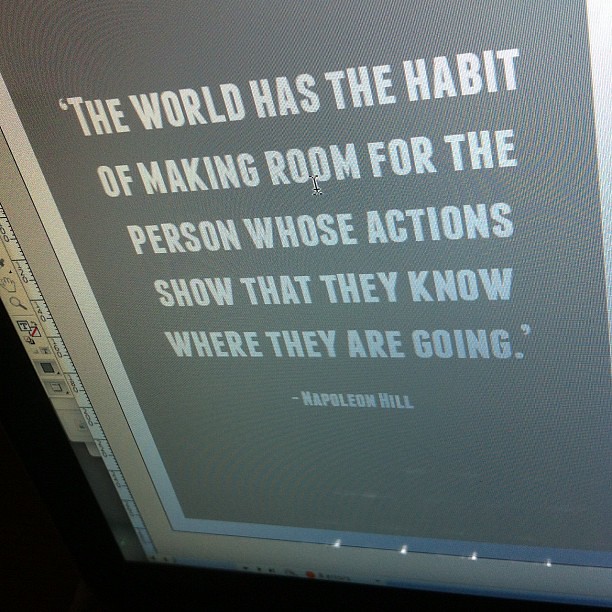The image depicts a computer screen, potentially a tablet or a monitor, displaying a design interface. The screen has a gray background and contains a variety of icons on a toolbar, including a magnifying glass, a move hand icon, and other graphic editing tools, positioned on the side. The image appears to be rotated 90 degrees from its intended orientation, creating a distinctive angle. Textured with wavy lines indicative of a photographed screen, the display features a bold white capitalized quote: "The world has the habit of making room for the person whose actions show that they know where they are going," attributed in smaller font to Napoleon Hill. This arrangement suggests that the screen is likely being used to design a printable sign, perhaps for a wall display.